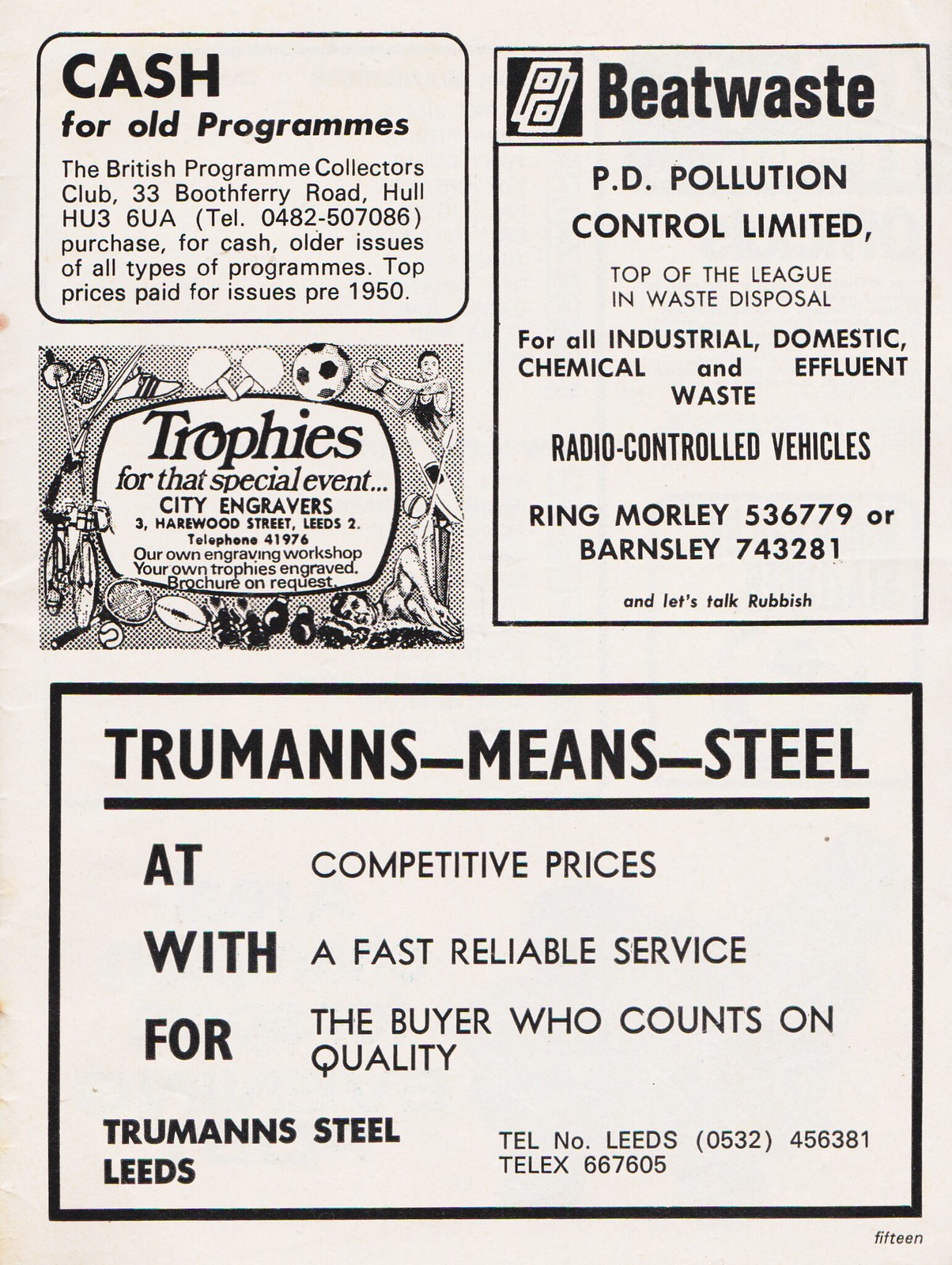This image depicts an aged, off-white page from a vintage game day magazine, specifically page 15. The rectangular page, taller than it is wide, is dominated by four well-spaced advertisements in black and varying shades of gray ink, suggesting significant discoloration due to age. 

In the upper left, an ad bordered with a black outline promotes "Cash for Old Programs" by the British Program Collectors Club, with the additional details of purchasing older issues pre-1950 for top prices at 33 Booth Ferry Road, Hull HU3 6UA. Contact number 0482-507086 is provided.

Directly below it, an ad framed with images of various sports equipment and athletes offers "Trophies for That Special Event" from City Engravers, located at 3 Harewood Street, Leeds 2. The advertisement highlights their in-house engraving workshop and brochures available upon request, alongside the telephone number 41976.

On the top right, an ad titled "Beat Waste" by PD Pollution Control Limited focuses on waste disposal services for industrial, domestic, chemical, and effluent waste. The header has a distinctive black square with white letters "P" and "D." The ad mentions radio-controlled vehicles and provides contact numbers for Morley (536-779) and Barnsley (743-281), underlining a slogan "Let's Talk Rubbish."

At the bottom of the page, a large ad with a bold black rectangular border declares "Truman's Means Steel," advertising competitive prices and fast, reliable service for quality-conscious buyers. Detailed contact information includes the telephone number (Leeds 0532) 456381 and telex number 667605, highlighting the company’s commitment to quality service.

The number 15 is subtly placed in the bottom right corner, indicating the page number. The style and layout of the page, along with its visual elements, clearly classify it as the advertisement section of an old magazine.